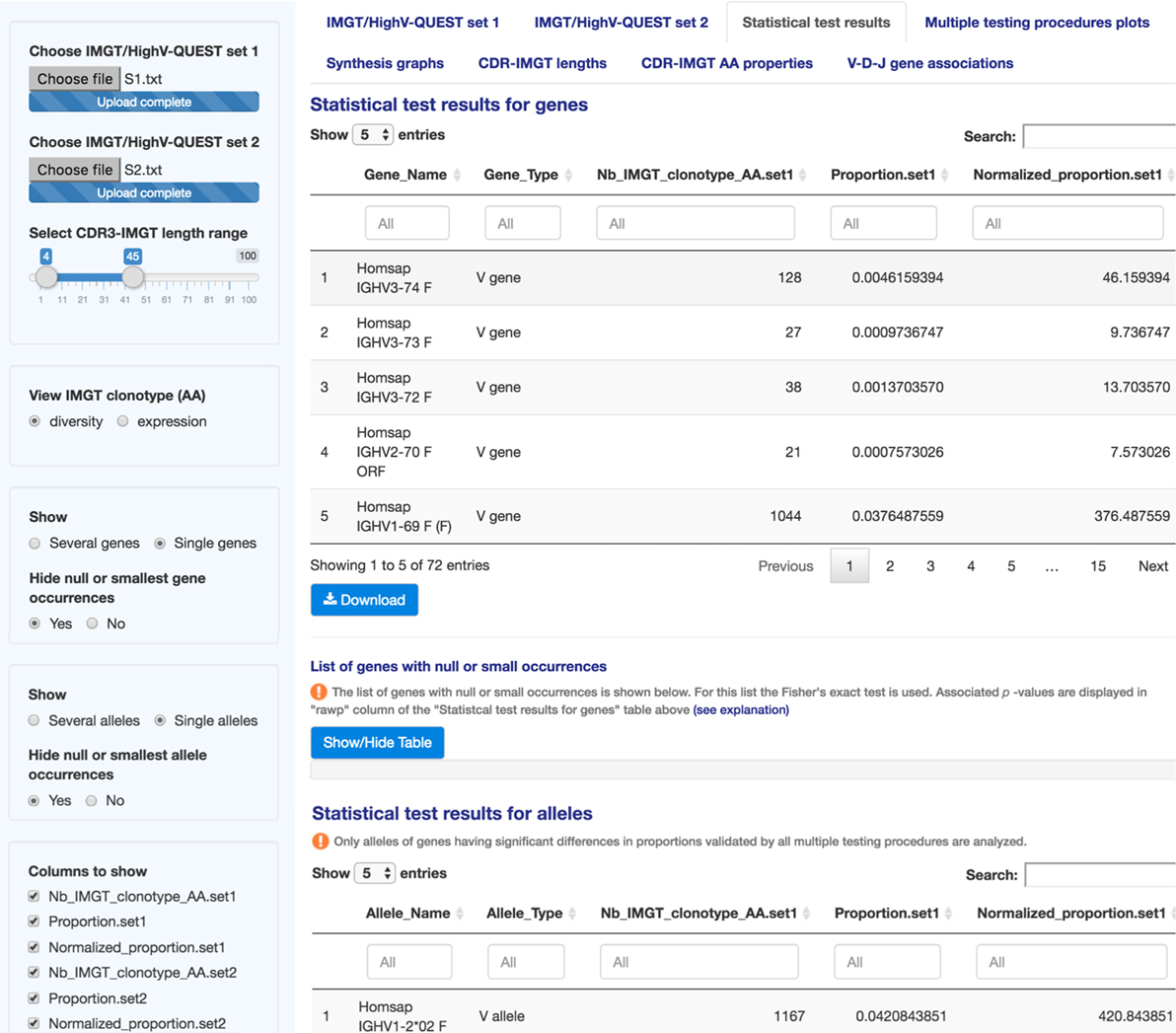**Detailed Caption:**

The image showcases a webpage dedicated to IMGT/HighV-QUEST, specifically opened to the "Statistical Test Results" section. The layout features two primary sections. On the left, there is a vertically elongated, light blue rectangle that provides an overview of IMGT/HighV-QUEST and details such as Set 1, Set 2, and length range. To the right of this, the majority of the page displays statistical test results in a structured, tabular format.

The results are presented in lists with multiple columns, each with a white background and entries in blue and black text. Gene results are prominently displayed in dark blue lettering. For instance, one result is detailed with a light gray background, featuring "HOMSAP IGHV3-7-4*04 F V gene" in black ink, followed by a numerical count of "128", several decimal values, and a percentage "46.159394". This format is consistent throughout the page, with numerous entries listed in a similar manner to provide comprehensive statistical data for IMGT/HighV-QUEST analysis.